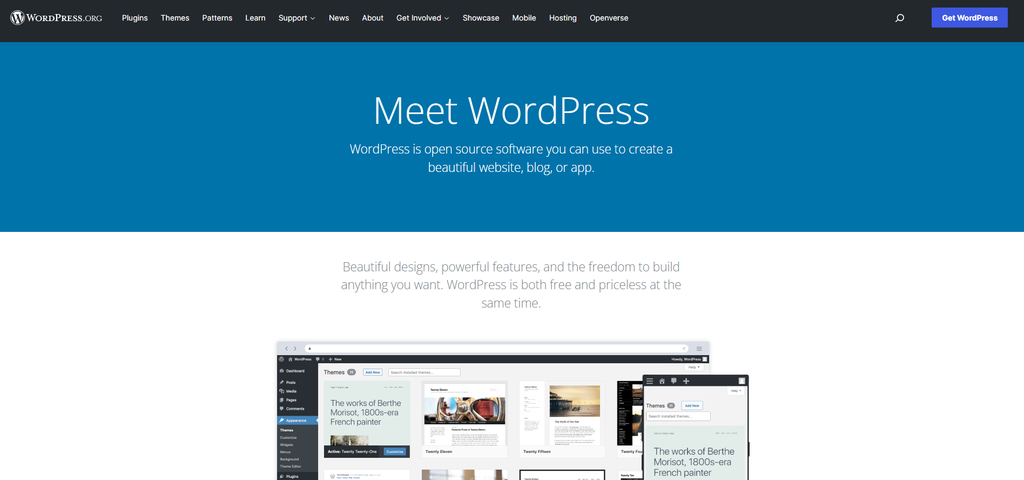The image is a screenshot of the WordPress.org homepage. The top navigation bar features options including 'Flights,' 'Themes,' 'Patterns,' 'Learn,' 'Support,' 'News,' 'About,' 'Get Involved,' 'Showcase,' 'Mobile,' 'Hosting,' and 'Operations.' In the top right corner, there is a prominent button labeled 'Get WordPress.' Centered on the page is the title 'Meet WordPress,' followed by a description: 'WordPress is open source software you can use to create beautiful websites, blogs, or apps. Beautiful designs, powerful features, and the freedom to build anything you want. WordPress is both free and priceless at the same time.' The focal point of the screenshot is an image displaying an open PC and a mobile device, showcasing a glimpse of the WordPress interface with various images and options visible on the screen. The interface suggests a user-friendly layout designed for creating and managing web content.